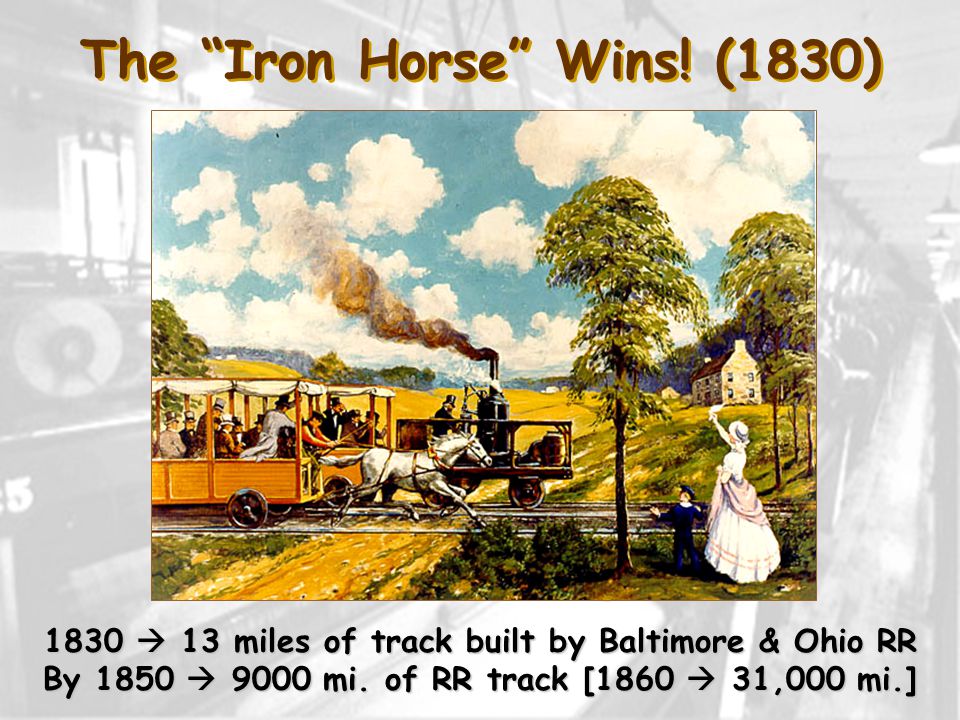This detailed color illustration, framed atop a light gray, black-and-white photographic background reminiscent of a factory interior, captures a dramatic race between a steam engine and a horse-drawn cart. At the top, the caption in vibrant red text with yellow shadowing declares, "The Iron Horse wins! (1830)." The main image, rectangular and inset within the larger background, showcases an old-fashioned steam engine on railroad tracks, outpacing a horse-drawn train. The right side of the image features a woman in a white dress and a young boy in a dark outfit, enthusiastically waving. This historical scene unfolds under a clear blue sky dotted with white clouds, with green trees and a house visible in the distant landscape. Below, black text caption notes, "1830 → 13 miles of track built by Baltimore and Ohio Railroad, by 1850 → 9,000 miles of railroad track, (1860) → 31,000 miles." The combination of color illustration and vintage graphic design encapsulates the evolution and rapid expansion of the early American railroad system.